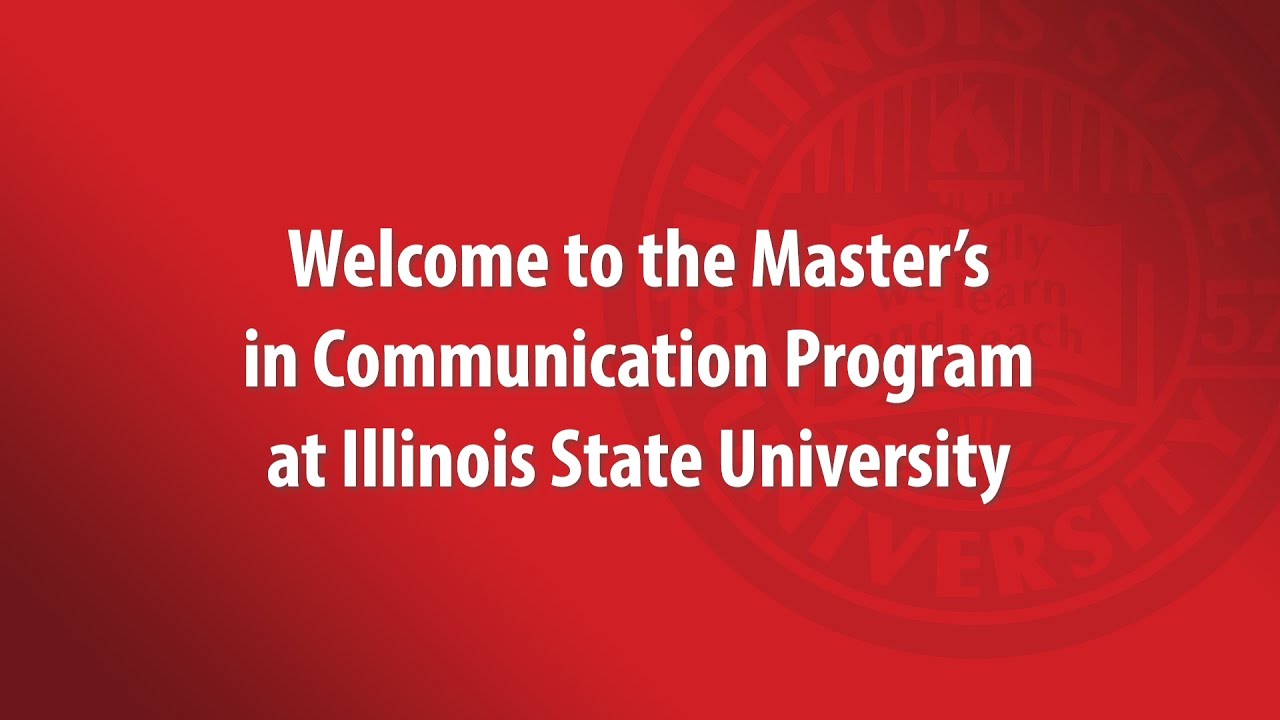A red gradient square features the official seal of Illinois State University. As the gradient progresses, it transitions to black in both the top right and bottom left corners. The seal is prominently displayed in the center, flanked by white text that reads "Illinois State University." The caption also includes a welcoming message, "Welcome to the Master's in Communication Program at Illinois State University."